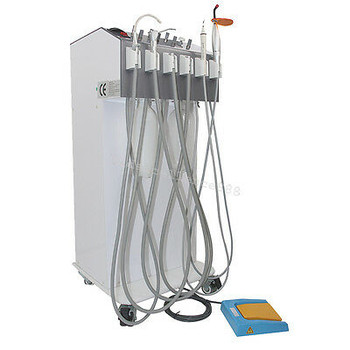The image depicts a professional-grade dental office equipment unit on a transparent background. The machine is a vertical, silverish-gray rectangular box with a pointed top and a flat base, wider at the bottom than the top. It has black wheels at each corner, making it portable. The unit features an array of dental tools, including a suction unit, a drill, and a UV light with an orange plexiglass shield used for applying sealants. These tools are connected to the device via several gray hoses clamped in white, horizontal clamps on the front. The top of the unit houses buttons, including a distinctive red and black one. Extending from the bottom is a blue-framed foot pedal with a yellow (tannish) pedal, used for controlling the drill's speed. The equipment appears pristine and well-organized, underlining its professional quality and functionality.